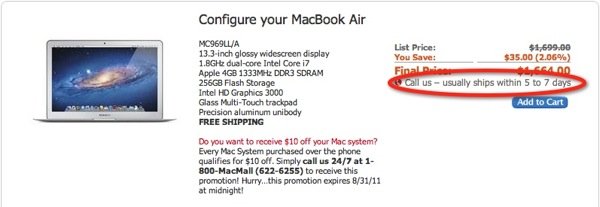The image displays a webpage dedicated to configuring and purchasing a MacBook Air. At the top center, the title "Configure Your MacBook Air" is prominently featured in black font. On the left-hand side, there is an image of an open MacBook Air laptop with a silver body. Its screen showcases a vivid blue sky with a circular arrangement of stars or light against a blue background.

Below the main title, key specifications of the laptop are listed, including a "13.3-inch glossy widescreen display." Following this, additional detailed information about the MacBook Air is provided.

Highlighted beneath the specifications, a promotional message in red offers a discount: "Do you want to receive $10 off of your Mac system?" This is accompanied by a descriptive paragraph and a contact phone number.

On the right-hand side, another column displays pricing details. The original list price of $1,699 is crossed out, indicating a discount. Below this, in red, it states, "You save $35, 2.06%." The final price is obscured by a red circle with the instruction "call us" within it. This red circle also mentions that the product "usually ships within five to seven days." At the bottom of this section, a blue "Add to Cart" button is available for customers ready to purchase.

The overall background of the image is white, emphasizing the information presented and ensuring clarity.